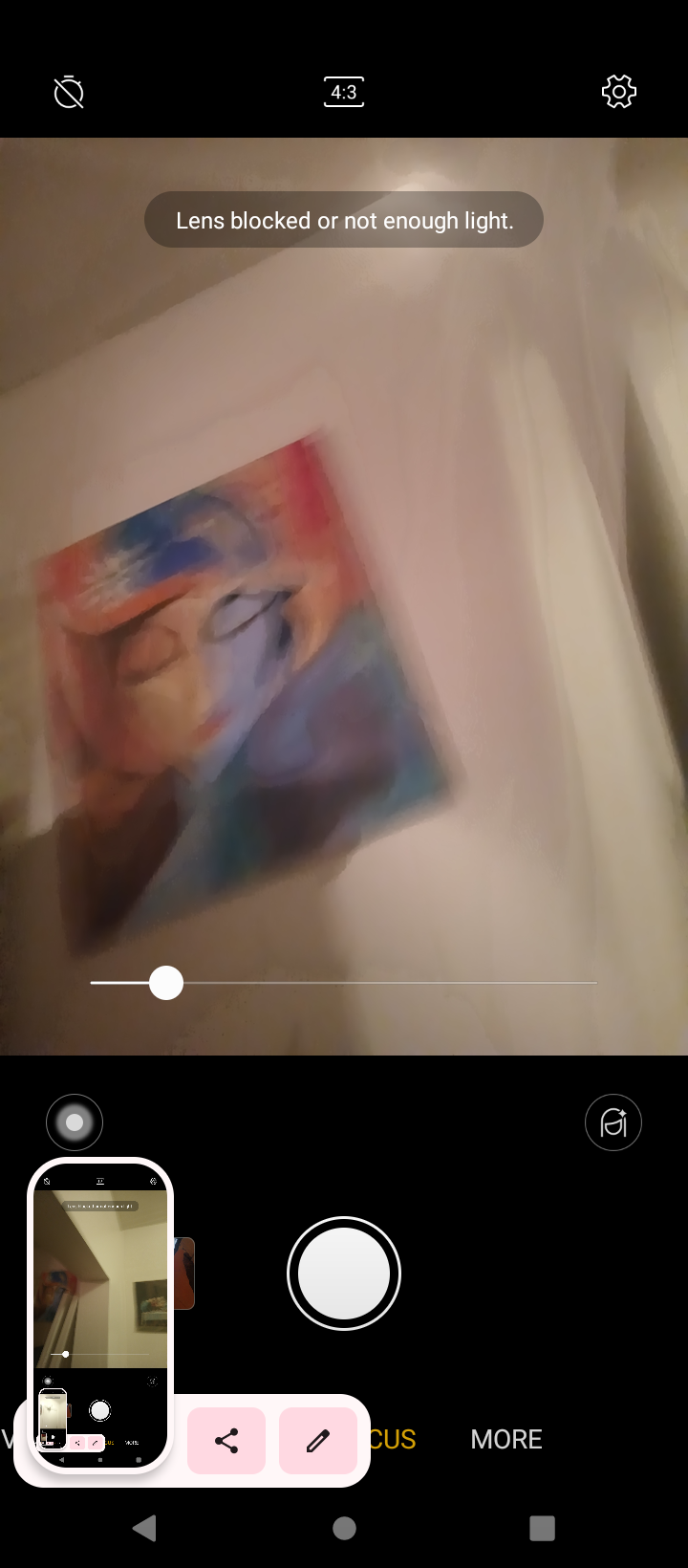The image shows a screenshot from an Android phone's camera app, captured while attempting to take a photo of a colorful painting of a woman with her eyes closed. The painting, which is slightly blurred, features a mix of pinks, blues, and yellows and appears to be on a white surface, possibly a door. The message "lens blocked or not enough light" is displayed at the top of the camera screen. The top portion of the image showcases three icons: a timer setting on the left, a 4:3 aspect ratio in the center, and a settings gear on the right. At the bottom, the phone's navigation buttons—a back triangle, a home circle, and a multitasking square—are visible, along with a white circle button for taking photos and a partially visible "more" button. In the lower left corner, there is a thumbnail of a previous screenshot. Overall, the screenshot captures the entire phone interface, including the camera functions and previous photo thumbnails, indicating an active photo-taking process while documenting a vibrant artwork.